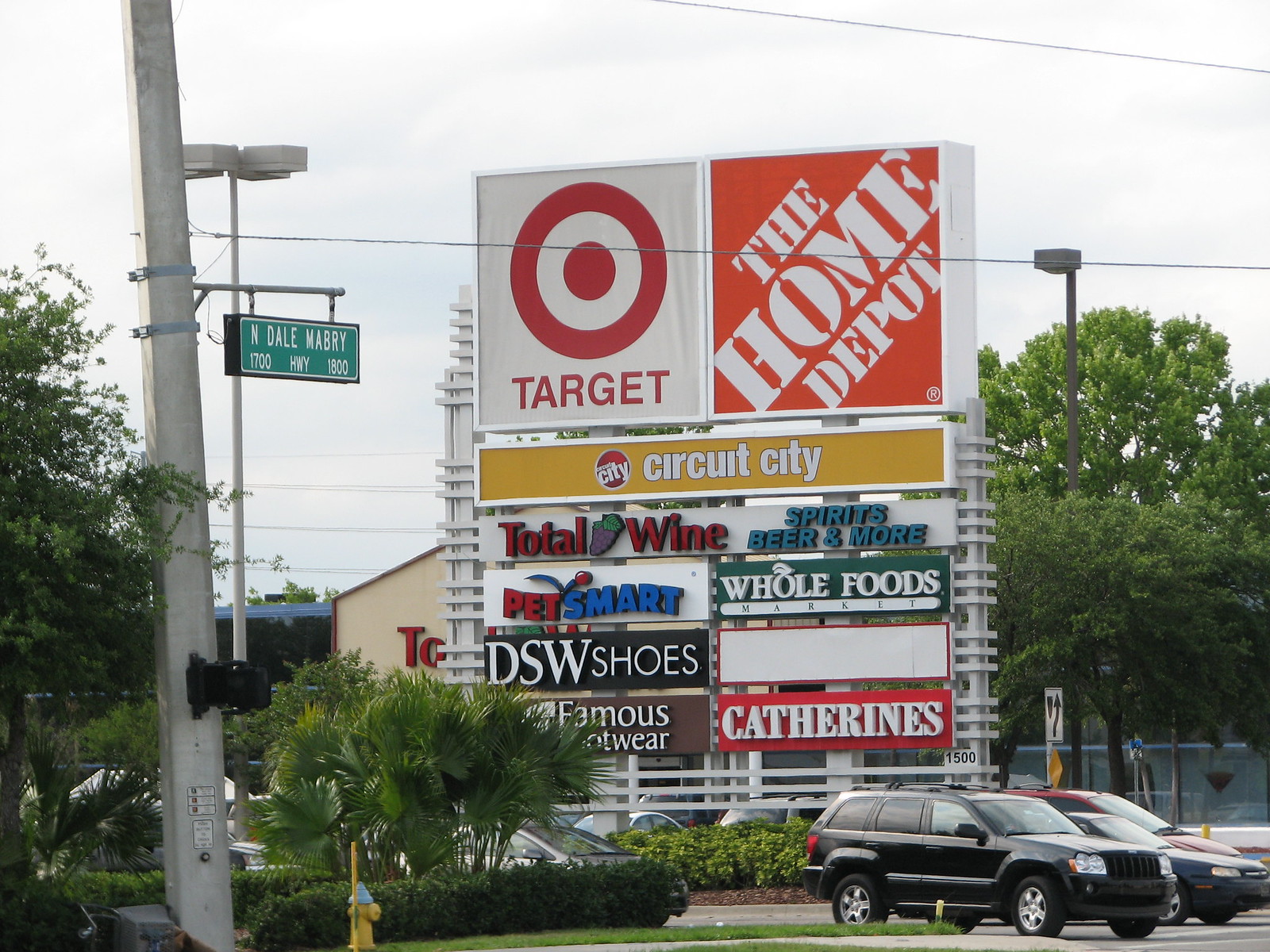The image captures a dynamic scene in front of a large shopping center sign filled with various store logos. Dominating the center, the sign lists several well-known stores including Target with its iconic red and white bullseye logo in the top-left, The Home Depot in white text against an orange background in the top-right, and Circuit City in white on yellow beneath them. Further down, the sign showcases additional stores such as Total Wine, Spirits, Beer, & More, PetSmart, Whole Foods Market, DSW Shoes, Famous Footwear, and Catherine's. The surrounding scene includes multiple cars leaving the shopping area, a tall green tree, and power lines crossing overhead. Flanking the sign, greenery and shrubs add a touch of nature with a yellow fire hydrant standing out on the left. The sky above is grayish-blue with some clouds. Additionally, a concrete post with a crossing light and an attached green and white street sign reads "N Dale Mabry Hwy 1600." To the left, a partially visible tan building with red text adds depth to the image.